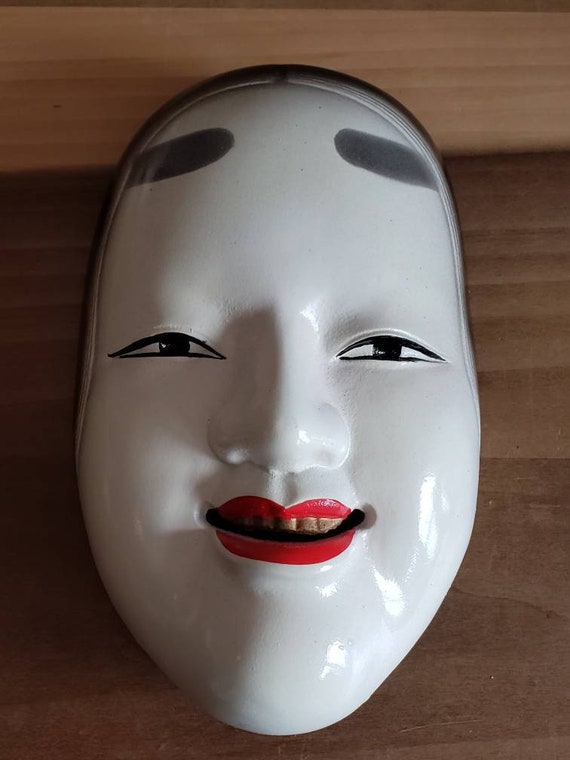The image depicts a close-up view of a traditional Japanese theater mask placed on a wooden surface. The mask has a distinctly ovular shape with a wide, chubby face, a large chin, and a high forehead. The face is painted white and features expressive details: elongated, narrow eyes with small black pupils, and painted eyebrows situated high on the forehead as large gray ovals. The mouth is adorned with prominent red lipstick, revealing golden teeth through a partially open smile. The nose is broad, complementing the other exaggerated facial features. The hair, painted flat against the head, parts in the middle. The wooden surface beneath the mask is brown with visible grain, and a large shadow partially covers both the surface and the mask, adding a dramatic effect to the scene. The overall clarity of the image is sharp, highlighting the intricate details of the mask and the texture of the wooden surface.